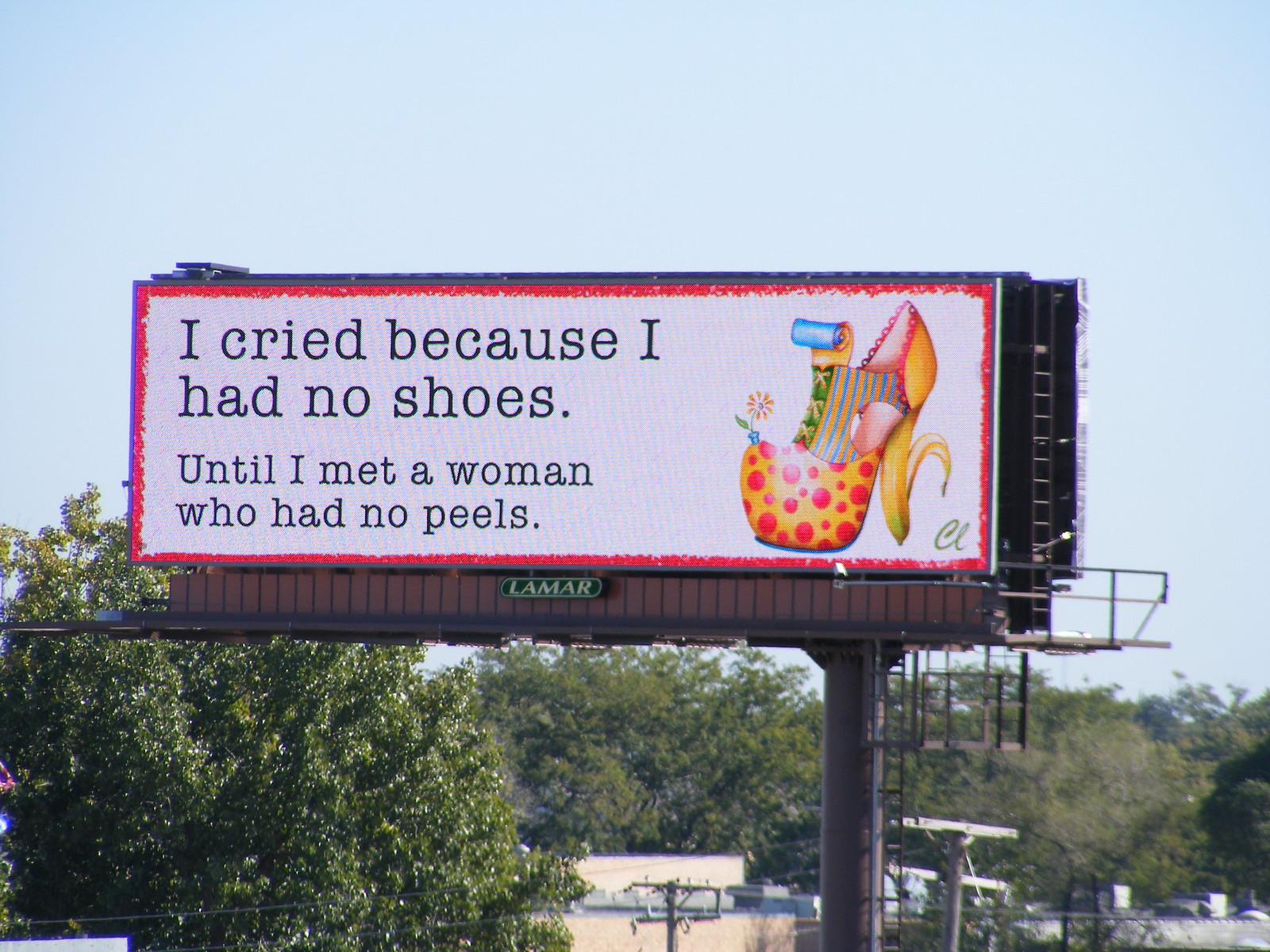The image shows a large rectangular billboard with a distinct red border, mounted on a singular six-cylinder metal pole. The billboard sits against a clear blue sky with no visible clouds, and features a ladder and walkway for maintenance access. It is situated in an outdoor setting with visible green trees, brown electrical poles, and some low brown buildings partially out of frame.

The billboard's background is primarily white, and in bold black text it states, "I cried because I had no shoes until I met a woman who had no peels." To the right of the text is an intricately designed, psychedelic high heel boot. The boot is highly colorful, reminiscent of the Beatles’ Yellow Submarine era, featuring a banana for the heel, peeling towards the front, and decorated with vibrant patterns including red polka dots on a yellow background, blue and orange vertical stripes, and an orange and blue roll-up shape. The tip of the boot is adorned with a red and yellow flower, complete with a green leaf and a blue pot. Additionally, the lower right-hand corner of the billboard displays the green text "CL."

At the base of the billboard, the brand name "Lamar" is displayed in white text within a green oval, indicating the company responsible for the billboard. The surroundings include trays in the ground and various electrical elements, contributing to the urban context of the image.